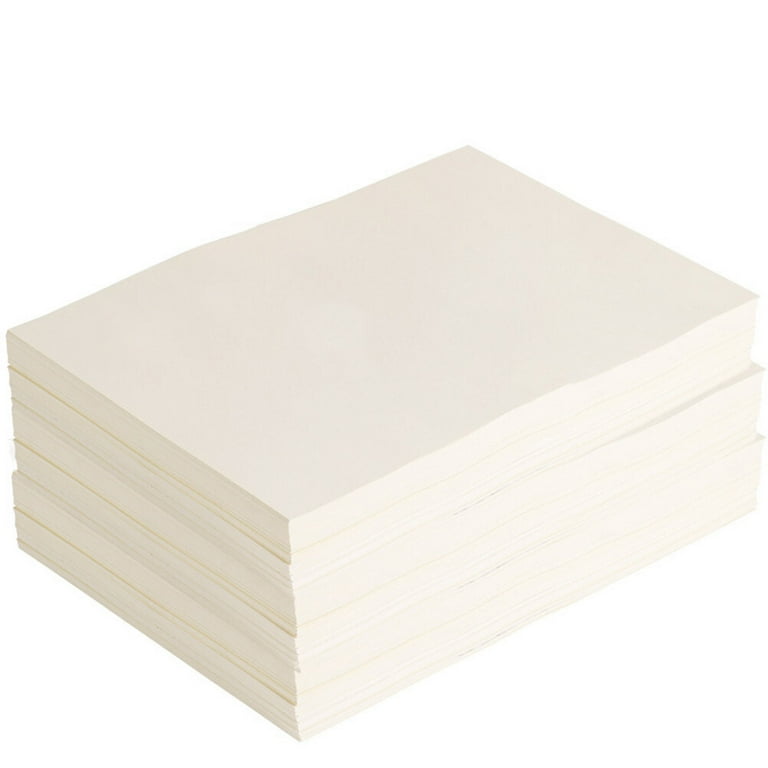The image depicts a product photo featuring a stack of what appears to be off-white or cream-colored paper, possibly printer paper or cardstock, set against a stark white background. The paper is arranged in three distinct, slightly offset stacks, giving a somewhat haphazard appearance yet maintaining a relatively straight alignment overall. The image is taken from an angle where the bottom of the stacks is to the left and extends upward to the right, allowing a clear view of the dimensions and the texture of the paper. One sheet in the middle appears thicker and more yellowish, potentially indicating a sticky base or core, suggesting these might be pads of sticky notes. Though mostly blank and rectangular-shaped, the sheets' placement and slight shadowing provide depth and a realistic perspective, emphasizing the product's tangible qualities as might be shown on an e-commerce website.